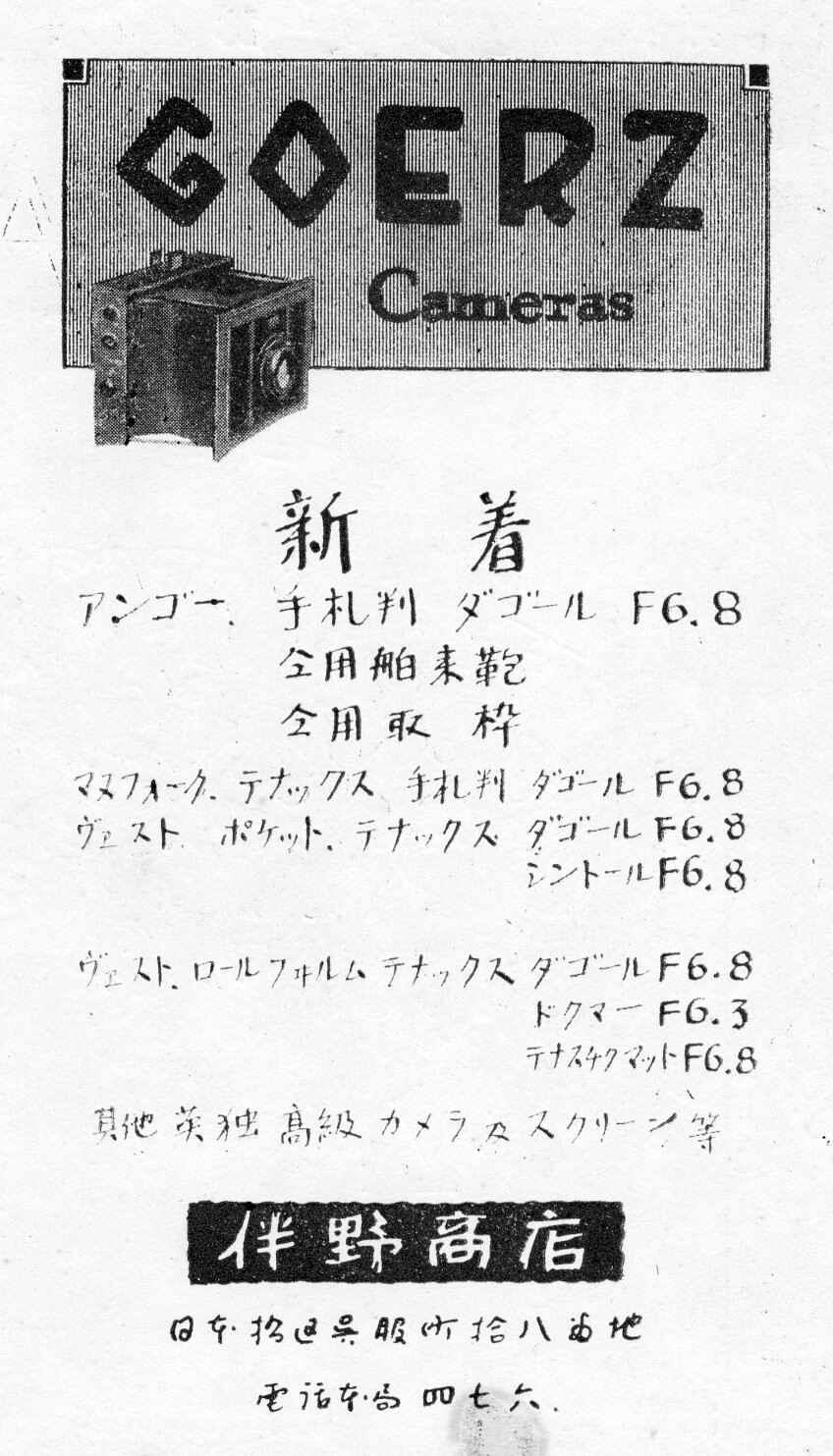The image depicts a vintage advertisement on a white background featuring a rectangular gray banner at the top. The banner is striped with white and contains the text "Goerz Cameras" in black font. Below the banner, there is a detailed drawing of an old-fashioned black box camera, reminiscent of early 1900s designs. The poster is densely populated with lines of text in Kanji, some of which end with numbers such as "f 6.8" and "f 6.3", repeatedly appearing throughout. Additionally, there is a black triangle with bold white Kanji characters. Overall, the ad melds historical photographic equipment imagery with extensive Asian script, making it a unique blend of cultural and technical elements.